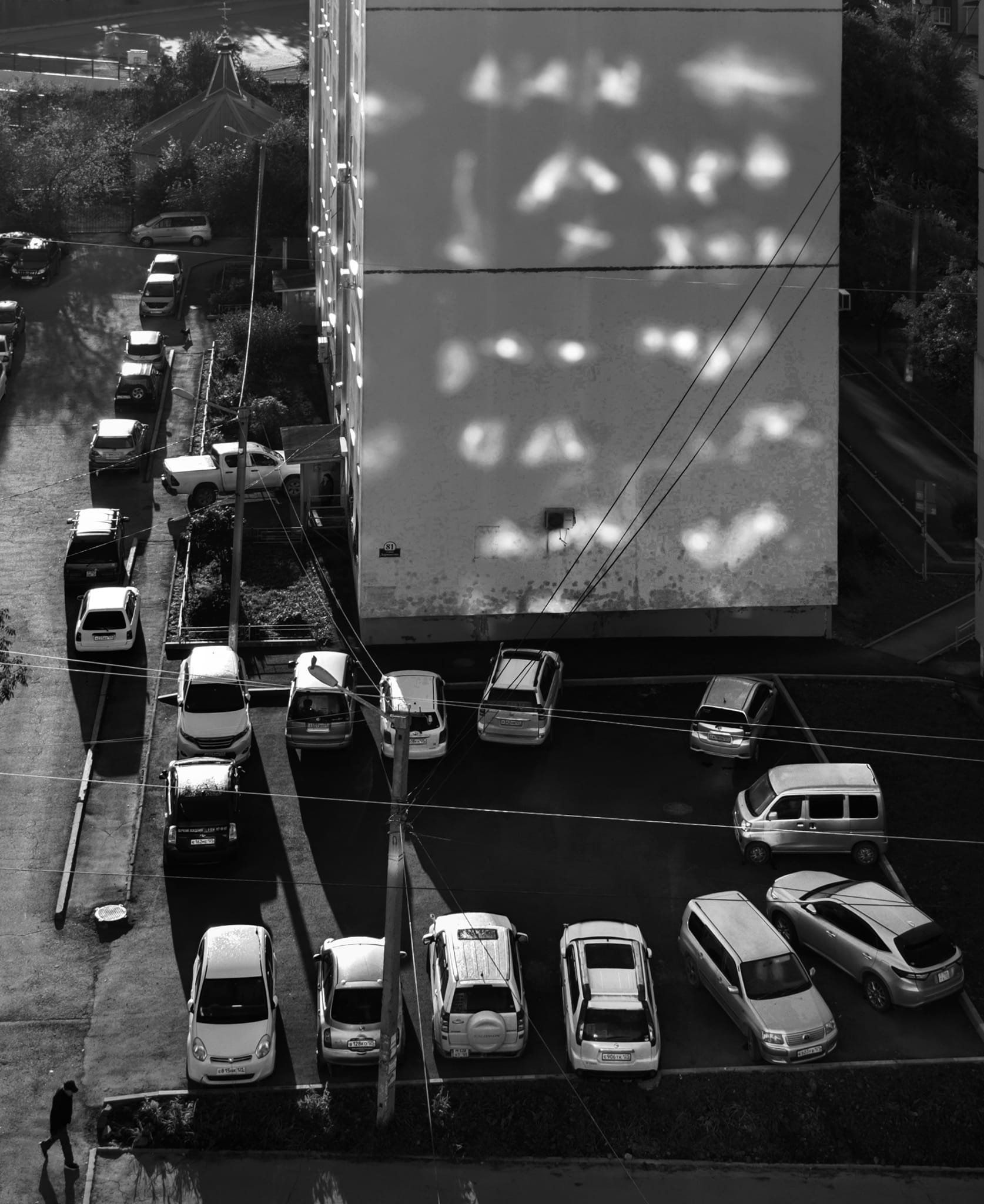In this black-and-white photograph, the viewer peers from a higher vantage point down onto a compact parking lot nestled beside a two-story concrete building, likely an apartment complex. The stark side of the building, devoid of windows, is illuminated by ambiguous reflections or lights, with shadow play suggesting the sun setting somewhere off-frame. Approximately 13 cars, appearing white or silver due to the monochrome filter, are parked in the lot and along a small adjacent street. The front of the building, partially visible at an angle, displays a small entrance and windows. The scene also captures a man in dark clothing and a hat walking at the bottom left of the frame, while a shadowy figure stands indistinctly in the doorway. In the background, trees and possibly a road or body of water add depth to the urban tableau.